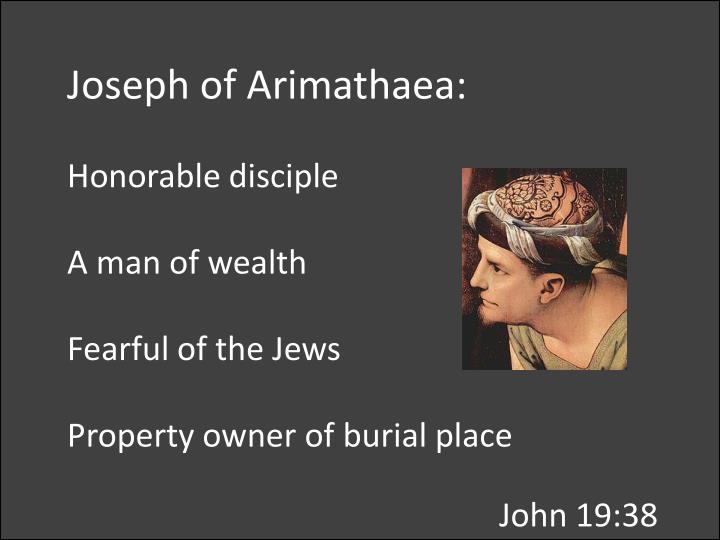The slide, part of a history presentation, features a dark gray background with white text detailing Joseph of Arimathea. At the top, the title reads "Joseph of Arimathea:" Following that, in a list format, it describes him as an "Honorable Disciple," "A Man of Wealth," "Fearful of the Jews," and "Property Owner of a Burial Place." To the right of this text is an image of a man presumed to be Joseph of Arimathea. He has brown hair and is pictured wearing an ancient hat with a scroll and floral pattern, likely painted or embroidered. He is dressed in a green outfit visible only from his shoulders up and is gazing to the left. Below the image, in the bottom right corner, the text "John 19:38" is displayed.